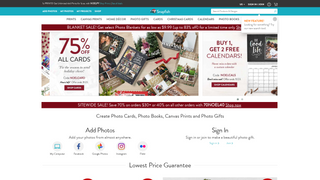This image depicts a shrunken view of a website. At the top of the page, there's a horizontal bar in a dark color—possibly black or brown. Below this, there is a lime green or mint green bar. Both of these bars contain labels or tabs that are too small to be legible.

On the right side of the green bar, there is a search bar. To the left of the green bar, there are additional symbols and clickable tabs. Further down the page, there are more tabs, sections, and categories designed for navigation and browsing the website, presumably for shopping.

In the center of the webpage, a pop-up advertises a sale, prominently stating, "75% off all cards." Below this, the promotion continues with "Buy one, get two free." Accompanying this text is an image displaying several cards.